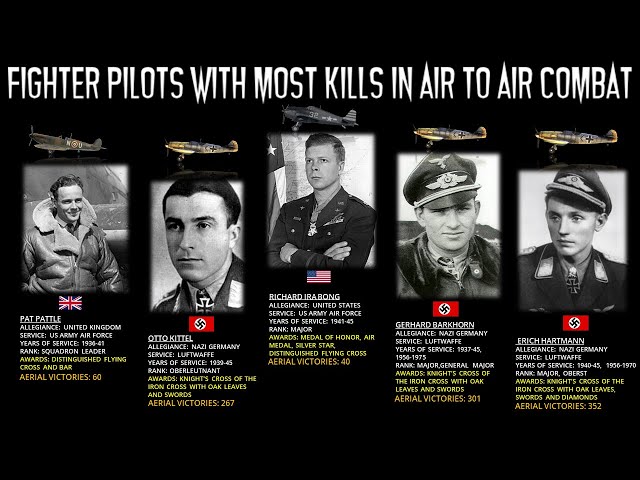The image is a detailed poster on a black background with white text titled "Fighter Pilots with Most Kills in Air-to-Air Combat." The poster features five pilots, each prominently displayed in black-and-white photographs beneath an image of the plane they operated during warfare. Below each pilot's image, their country's flag is showcased, followed by comprehensive details including their name, allegiance, years of service, rank, awards, and total aerial victories, which range from 60 to 352.

The pilots listed are Pat Paddle from Great Britain, Otto Kittel from Nazi Germany, Richard Bong from the United States, Gerard Barkhorn from Nazi Germany, and Eric Hartmann from Nazi Germany. The textual information on the poster varies in color, with most details in white and some descriptions highlighted in yellow. Notably, the pilots from Nazi Germany have the highest kill counts, emphasizing their prominence in the list.